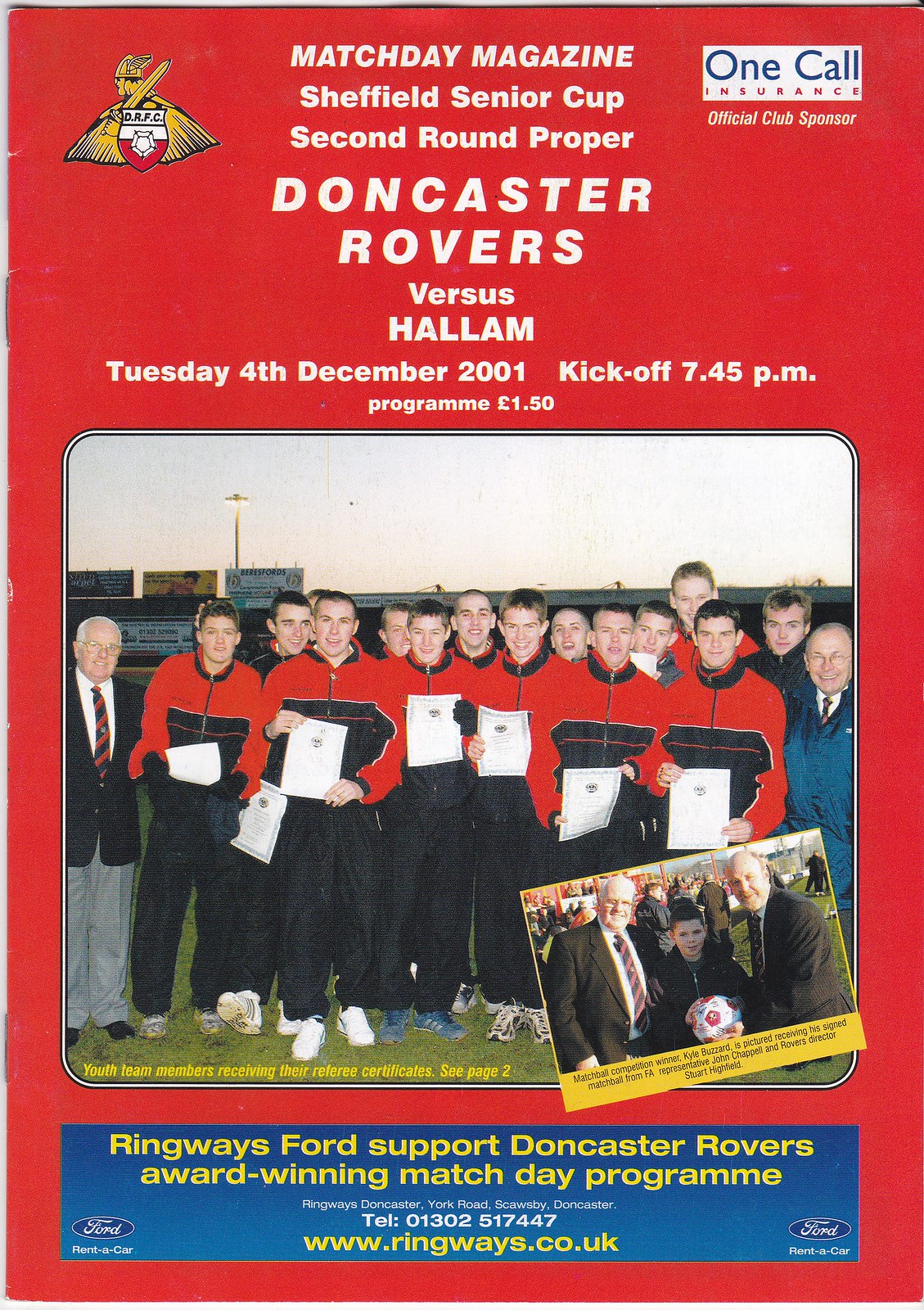In the center of the image, we see a group of young men in red jackets and black pants, standing in a grassy field, flanked by a few official-looking men, one of whom is elder and dressed in a suit and tie. Surrounding this central photograph, there is a red background with detailed text in lighter colors. At the top, it reads, "Match Day Magazine, Sheffield Senior Cup 2nd Round Proper, Doncaster Rovers vs. Hallam, Tuesday, 4th December 2001, Kickoff, 7.45pm." Below that, in smaller font, it notes, "Program £1.50." Additionally, there’s a blue highlight at the bottom with the text, "Ring Rovers for support - Doncaster Rovers award-winning Match Day Program," along with a website and telephone number. The overall style and details suggest this is a program cover for a football match that took place in the early 2000s. The color palette includes red, white, black, blue, and yellow, contributing to a visually striking design.